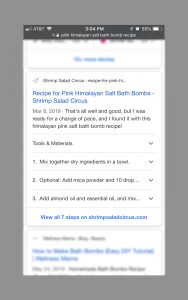This screenshot, captured at 3:14 PM with 88% battery life on an AT&T network, showcases a search bar containing the query "pick handyman." The gray-background interface reveals the results under a heading that reads "Pink Himalayan Salt Bath Bombs Recipe." Below this title, the webpage provides detailed sections on tools and materials required to create bath bombs, as well as step-by-step instructions, numbered from 1 to 3. Additionally, the webpage features related recipes and articles, such as shrimp salad and circus-themed content.